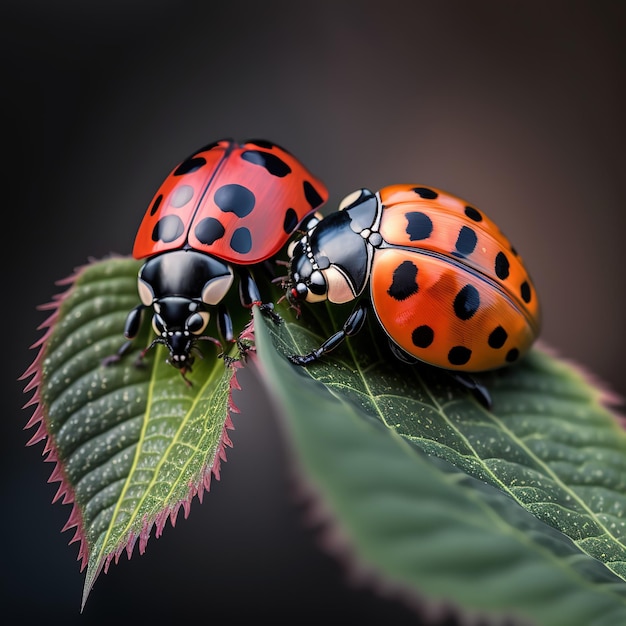The image depicts a dark, almost black background that accentuates two overlapping leaves, each hosting a ladybug. The leaf on the left is smaller, deep green with purple-like jagged edges, and distinctly outlined. Resting on it, a ladybug with a dark red shell and black body faces towards the viewer, showcasing its three-segmented head with black dots that are irregularly placed, and white eyes. The right leaf, nearly twice as large and similar in green coloring but with prominent yellow streaks and blurred edges, hosts a larger ladybug. This ladybug has an orangey-red shell, divided into visible segments, appearing wider than its counterpart. It faces the left, providing a side view of its body and a clear sight of its identical black head with white eyes. The overall composition highlights the contrast between the ladybugs' colors and their respective leaves, all set against a muted dark backdrop.